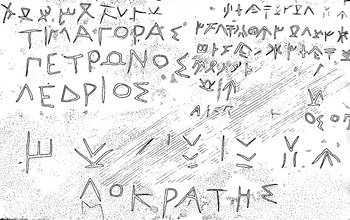The image appears to be an intricate etching or a pen and ink drawing, rendered entirely in grayscale. It depicts a complex array of characters and symbols, resembling a blend of ancient scripts and hieroglyphics. While the precise meaning of these characters remains unclear, the composition suggests a historical or archaeological context, as though it were an ancient artifact or a journal page filled with hybrid glyphs. The left and lower portions of the image seem to feature what might be Greek-like writing, while the upper right-hand section is dominated by hieroglyphic symbols of varied shapes and sizes. The overall presentation is somewhat chaotic and seems more suited to a depiction of cave art or an ancient script found on a wall, rather than neatly organized text on paper or parchment. The entire piece is executed with a low level of precision, making it difficult to discern finer details, but it evokes the feel of something one might find in a museum, like a relic from a bygone era.